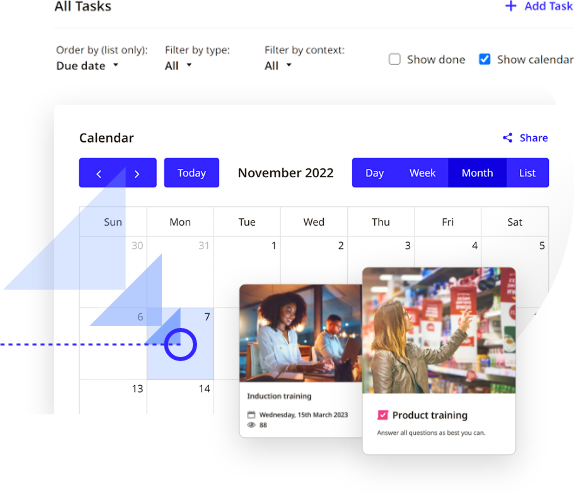This detailed caption describes an image featuring a comprehensive, interactive organizational tool, focusing particularly on its calendar view and task management interface:

---

The image showcases a detailed view of an organizational tool's interface, primarily emphasizing the calendar and task management features. In the top right corner, there is a prominent blue plus sign symbolizing the addition of new tasks. The tasks are displayed with blue text and are organized by list only, with sorting options available by due date. Filters are also provided by task type and context, alongside options to show completed tasks, display a calendar view, and a blue check mark to verify completion.

The calendar is positioned prominently, with navigation tools on the right side including buttons for sharing, left and right arrows to navigate between dates, a 'Today' button to return to the current date, and a dropdown to select the view between 'Day,' 'Week,' 'Month,' or 'List.' The calendar displays the days from Sunday to Saturday, starting from the 30th of one month and moving through the 31st to the 1st of the next month, continuing to the 7th, where a highlighted dash mark appears on the 7th.

Within the calendar grid, notable elements include circled dates and triangles increasing in size going to the left, indicating specific events or deadlines. To the right, there's a sidebar with an entry titled "Induction Tray," dated Wednesday, March 15th, 2023, showing that it has been viewed multiple times. Accompanying images depict a person working on a computer in an office and a woman examining products in a store. A red check mark with a note instructs to "Answer all questions as best you can," indicating it's related to product ratings or reviews.